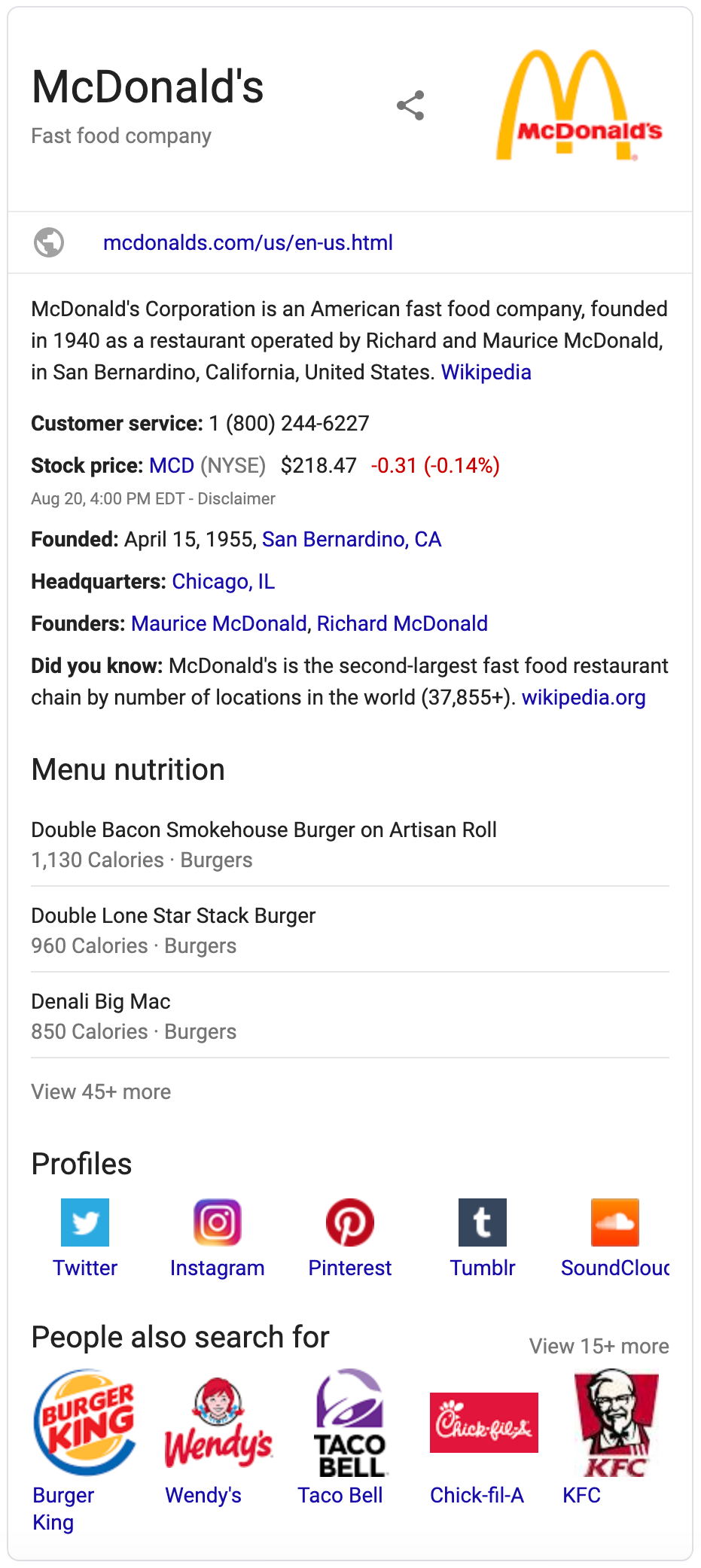This image showcases various elements related to McDonald's, the globally renowned fast-food company. Prominently featured are the iconic golden arches and the McDonald's name, situated in the upper right-hand corner of the image. A URL is included, directing to "mcdonalds.com/US/EN-US.html" for further information.

The image also provides a brief historical overview, noting that McDonald's Corporation is an American fast-food entity founded as a restaurant on May 15, 1940, by Richard and Maurice McDonald in San Bernardino, California. Additional historical context is given, indicating the company's official corporation date was April 15, 1955, with its current headquarters located in Chicago, Illinois.

Further details include a customer service contact number (1-800-244-6227) and financial data, noting a stock price of $218.47, which is down by 0.31 as of August 10th at 4 p.m.

A "Did You Know?" section highlights that McDonald's is the second-largest fast-food chain worldwide by the number of locations. This part of the image refers viewers to Wikipedia for more detailed information.

Additional content features a food menu with nutritional information, listing items such as a Double Bacon Cheeseburger Smokehouse Burger on an artesian roll with 1130 calories, a Double Lone Star Stack Burger with 960 calories, and a Denali Big Mac with 850 calories.

Social media profiles linked from the image include Twitter, Instagram, Pinterest, Tumblr, and SoundCloud. Competitor profiles mentioned include KFC, Chick-fil-A, Taco Bell, Wendy's, and Burger King.

This comprehensive image encapsulates McDonald's history, menu offerings, social media presence, and more, providing a thorough snapshot of the fast-food giant.